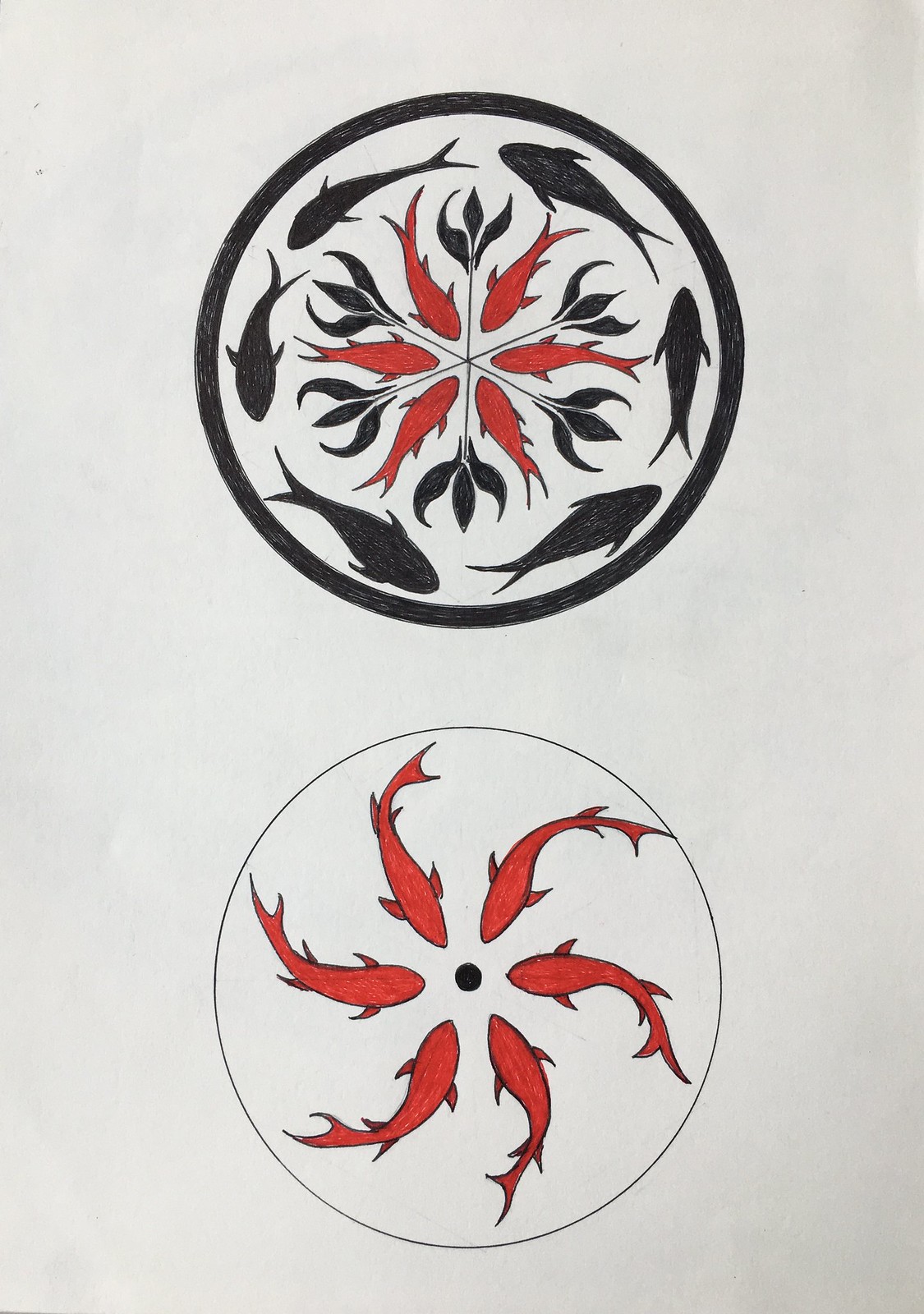This image showcases an intriguing drawing with a yin-yang inspired design. At the bottom, there is a meticulously drawn, perfect circle with a dot precisely centered within it. Surrounding this central dot are six vibrant orange koi fish, each gracefully swirling towards the circle's heart, creating a visually captivating pattern. Above this section, the drawing features the same configuration of koi fish, but this time depicted in contrasting black. These black koi fish encircle their orange counterparts, augmenting the sense of balance and harmony characteristic of the yin-yang motif. The intricate arrangement and fluid motion of the fish add depth and complexity to the artwork, making it a visually striking and thought-provoking piece.